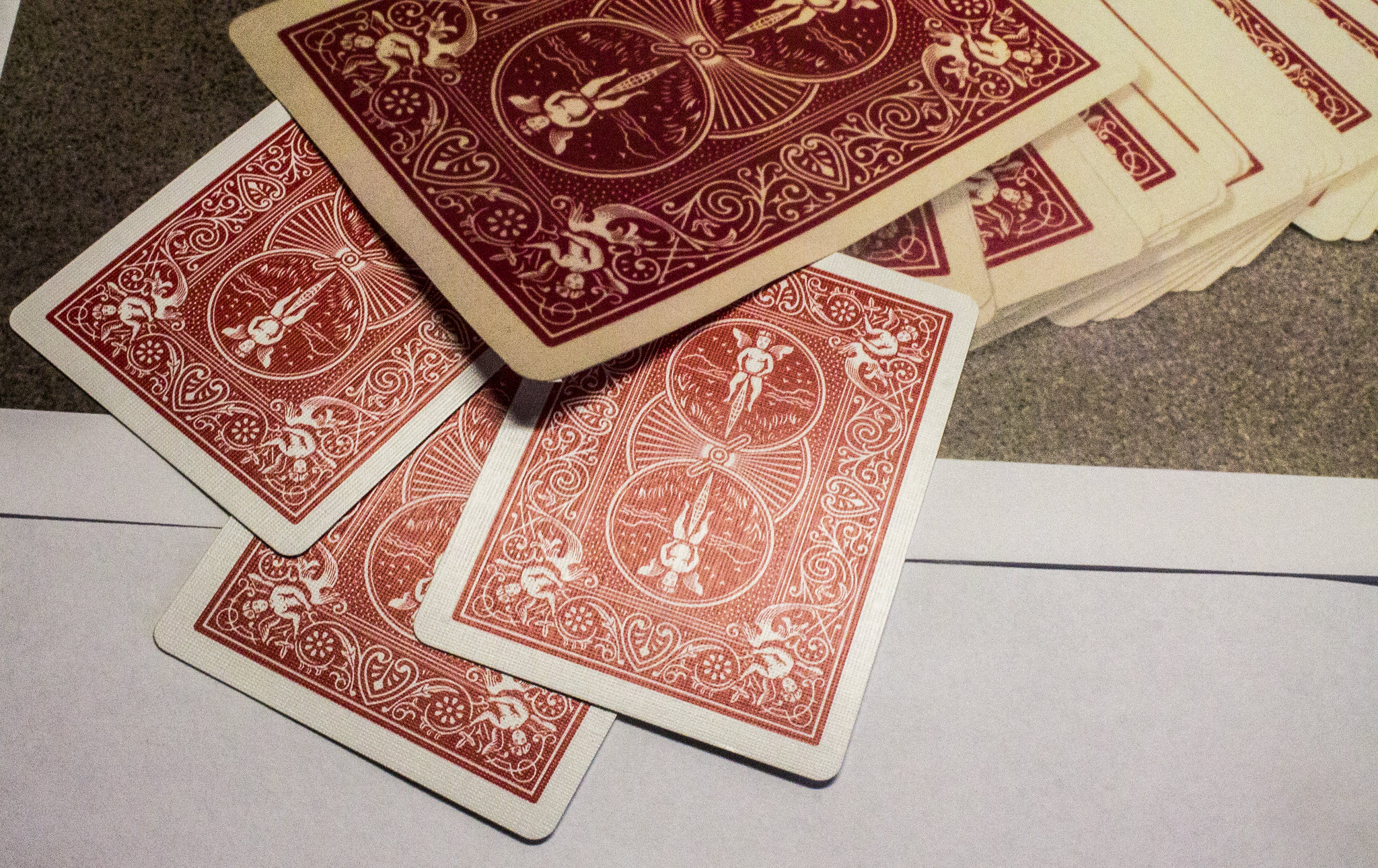A close-up photograph captures an array of vintage playing cards, scattered across what appears to be a grayish-brown carpet, resting beside a white countertop. The edges of the cards show a distinct yellowing, indicative of their age, with the top card exhibiting a slight bend. This top card, predominantly dark red with ivory accents, portrays intricate designs featuring angelic figures with a single pair of wings, surrounded by elaborate arabesque patterns. The surrounding cards, lighter shades of red with stark white contrasts, echo the same ornate patterns. Each card's back is richly detailed, showcasing hearts, flowers, and arabesque motifs, but none reveal their face values or suits, maintaining an air of mystery.